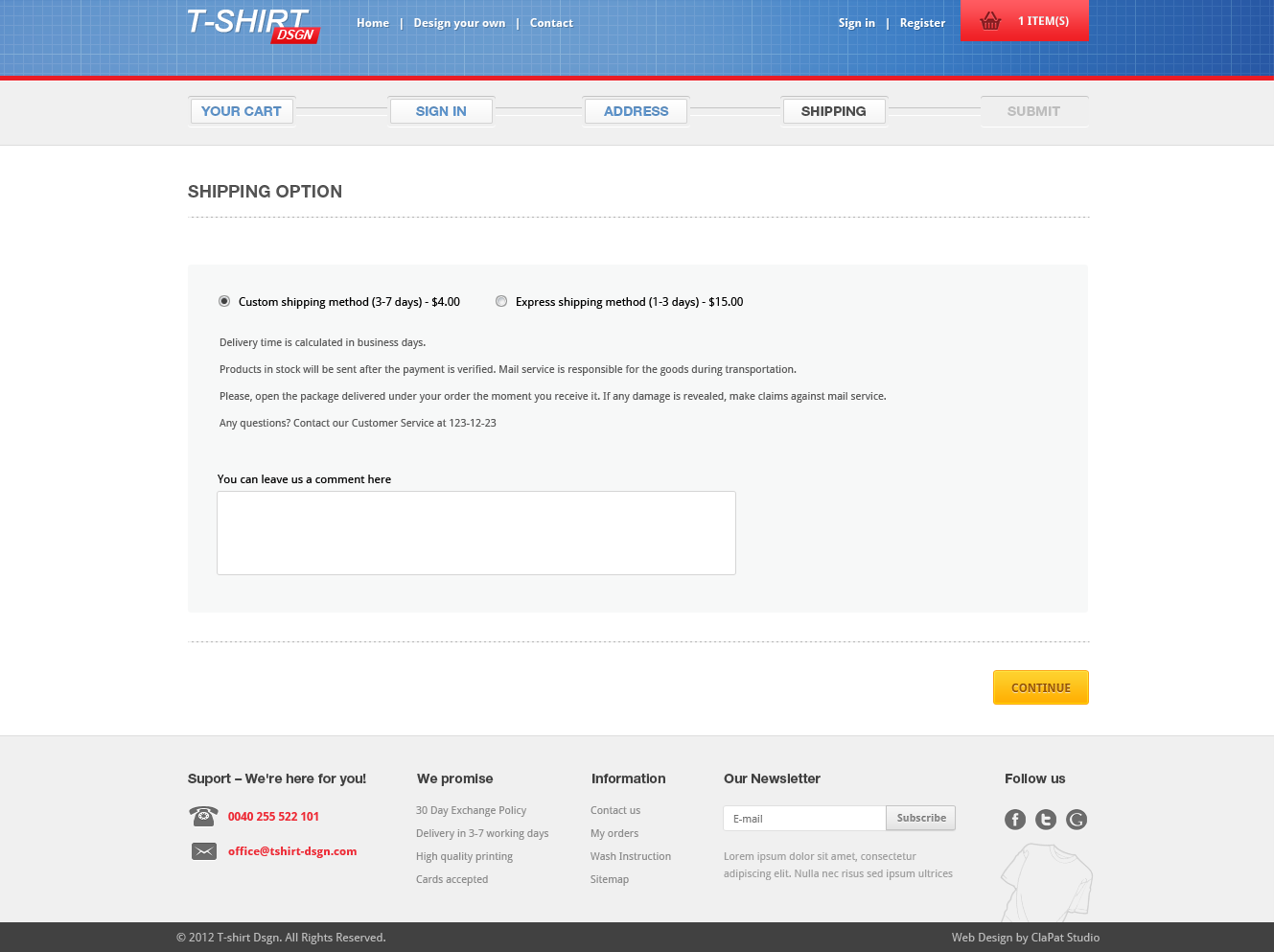At the top of the image, there is a gradient border that transitions from light blue on the left to dark blue on the right. This border also features a delicate grid pattern. On the left side, the word "T-SHIRT" is prominently displayed in capitalized, italicized white letters. Positioned just below this is a small red banner at the bottom right that reads "DSGN" in white text.

Beneath these elements, there are three menu options in small white text: "Home," "Design Your Own," and "Contact." These options are separated by small white divider lines, one following "Home" and another after "Design Your Own." On the right side of this section, a bold white "Sign In" option is visible, followed by another small white divider, and then the word "Registered."

Below this, a progress bar or menu is presented. It includes the stages: "Your Cart," "Sign In," "Address," "Shipping," and "Submit." The first three stages ("Your Cart," "Sign In," and "Address") are in bold blue font. "Shipping" is in bold black, indicating the current stage, and "Submit" appears in light gray, denoting that it is disabled.

Underneath this section, there is a white background with the words "SHIPPING OPTION" in capital black letters. A light gray line divider follows. Then, within a rectangular area with a light gray background, two shipping options are provided in small black bold text. The first option, "Custom Shipping Method (3-7 days) - $4," is selected, indicated by a black dot in the middle of the selection circle. To the right, the unselected option says "Express Shipping Method (1-3 days) - $15."